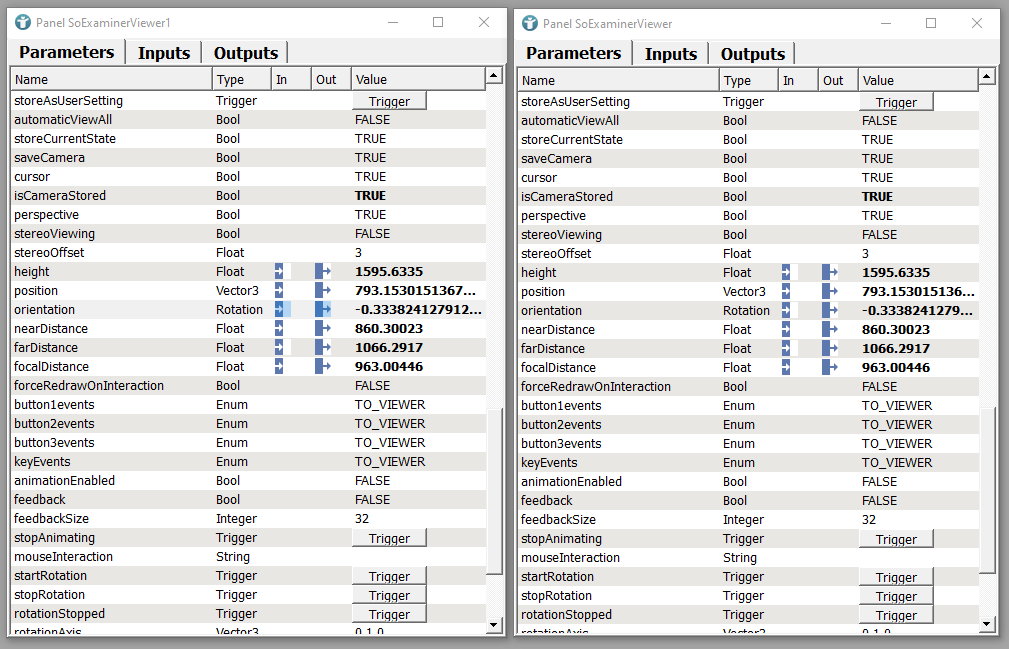The screenshot captures two juxtaposed screens within a highly technical application interface. The interface is partitioned into three tabs located at the top, labeled "Parameters," "Inputs," and "Outputs." Below these tabs, a comprehensive list of technical settings spans the view. The settings displayed from top to bottom are:

- Stores User Setting
- Automatic View All
- Store Current State
- Save Camera
- Cursor
- Is Camera Stored
- Perspective
- Stereo Viewing
- Stereo Offset
- Height
- Position
- Orientation
- Near Distance
- Far Distance
- Focal Distance
- Force Redraw on Interaction
- Button One Events
- Button Two Events
- Button Three Events
- Key Events
- Animation Enabled
- Feedback
- Feedback Size
- Stop Animating
- Mouse Interaction
- Start Rotation
- Stop Rotation
- Rotation Stopped
- Rotation Axis

Both screens display identical columns of settings, suggesting that they may represent different versions or states of the same application configuration. Additionally, certain settings such as "Height," "Position," "Orientation," "Near Distance," "Far Distance," and "Focal Distance" feature blue arrows to the right, indicating associated numerical values. This meticulous array of parameters likely pertains to detailed adjustments within a computer application, potentially for purposes such as user interface customization, camera configuration, or interactive animation setup.